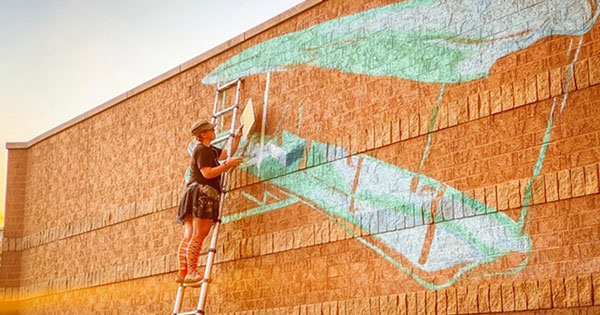In the photograph, a woman is captured mid-action as she paints a large, towering brown brick wall outdoors. The wall, made of brown stone bricks, features three distinct horizontal lines where the bricks protrude slightly. The artist stands midway up a ladder, balancing a square piece of paper and a paintbrush in her hands. Splashes of light green, white, and brown paint already adorn the wall, hinting at an ongoing mural. She is dressed in a brown hat, black t-shirt, black skirt, and conspicuously tall orange socks, with a tan fanny pack around her waist and a watch on her wrist. The day appears overcast, with a sky painted in shades of gray and white. The design on the wall remains somewhat unclear, but it suggests interconnected shapes that could be reminiscent of slides.